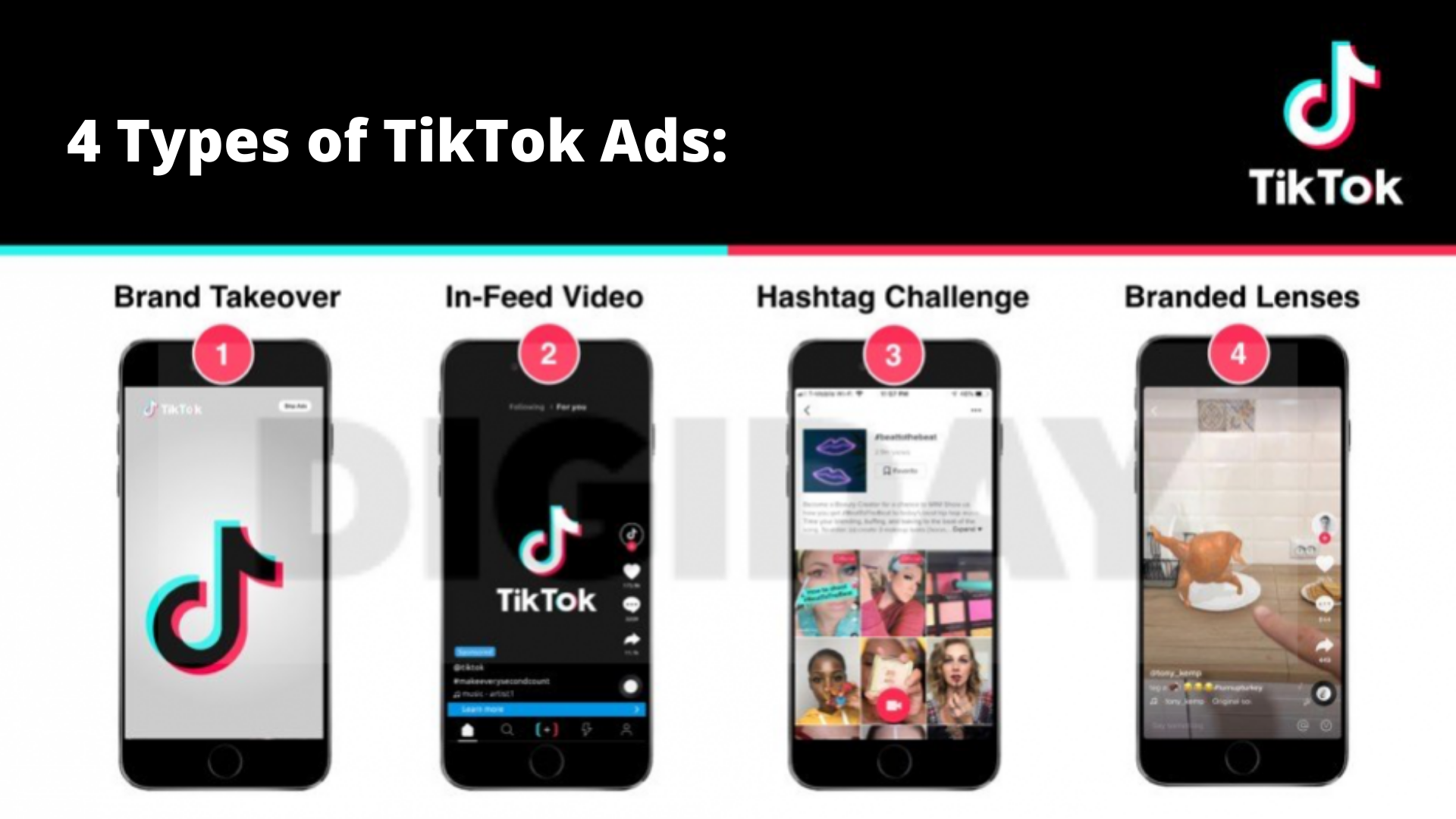The advertisement presents four types of TikTok ads, organized in a structured, visually distinct layout. The ad itself is divided into two main sections. 

The upper portion features a black rectangular background with the phrase "Four Types of TikTok Ads" boldly written in white text. To the right of this title is the recognizable TikTok logo, complete with the signature music note.

The body of the ad transitions to a clean white background, punctuated by black text and a series of four images, each portraying a different type of TikTok ad. Each image is accompanied by a red circle with a corresponding white number (from one to four), positioned above to indicate its sequence.

1. **Brand Takeover**: This section features a picture of a cell phone displaying the TikTok logo, highlighted with a red circle containing a white number one.
2. **In-Feed Video**: Here, a cell phone screen is shown with the TikTok logo set against a black background, accompanied by the familiar TikTok controls.
3. **Hashtag Challenge**: This depiction includes a series of squares containing images of influencers, signifying the participatory and community-driven nature of hashtag challenges.
4. **Branded Lenses**: The final image features a cell phone showcasing a virtual interface that allows users to overlay virtual objects onto their environment, illustrating the interactive aspect of branded lenses.

Through these detailed visuals, the ad effectively communicates the variety of advertising options available on TikTok, each tailored to engage users in unique and interactive ways.